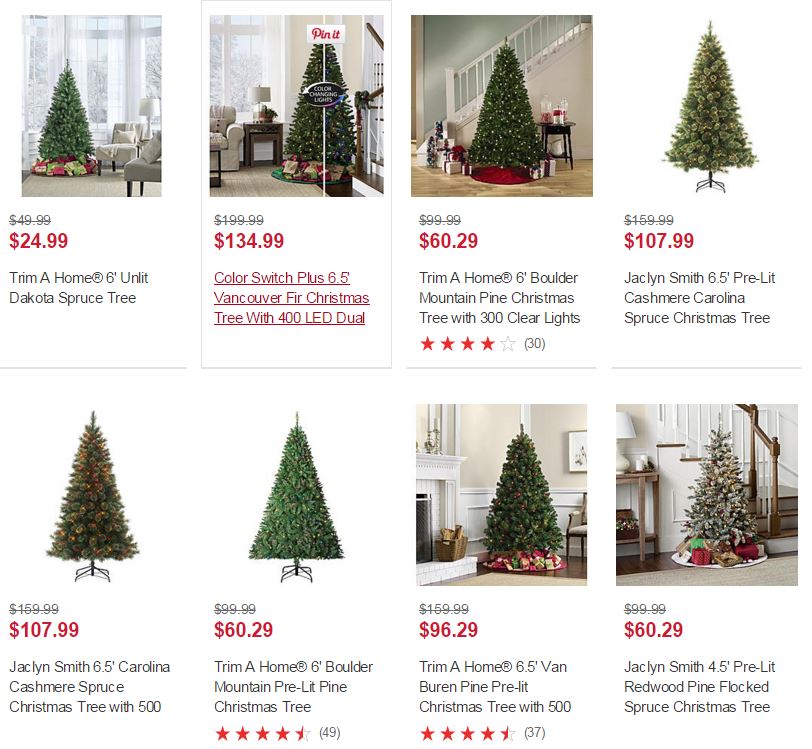The image displays four different Christmas trees, each accompanied by their names, prices, and descriptions. Most trees are situated indoors, adorned with festive decorations and presents, while some images are stock photos featuring a traditional Christmas tree setting. The detailed breakdown of each item is as follows:

- **Top Left:** Originally priced at $49.99, now available for $24.99. This is a Trim A Home 6-foot unlit Dakota Spruce Christmas tree.
- **Top Right:** Previously listed at $199.99, now reduced to $134.99. This model is a Color Switch Plus 6.5-foot Vancouver Fir Christmas tree featuring 100 LED dual lights.
- **Bottom Left:** Initially $99.99, now priced at $60.29. This is a Trim A Home 6-foot Boulder Mountain Pine Christmas tree, equipped with 300 clear lights and holding a four-star review with 30 ratings.

Visually, each tree showcases its unique aesthetic, with some emphasizing their unlit natural look and others highlighting their pre-lit convenience, all set against cozy, decorated home interiors.